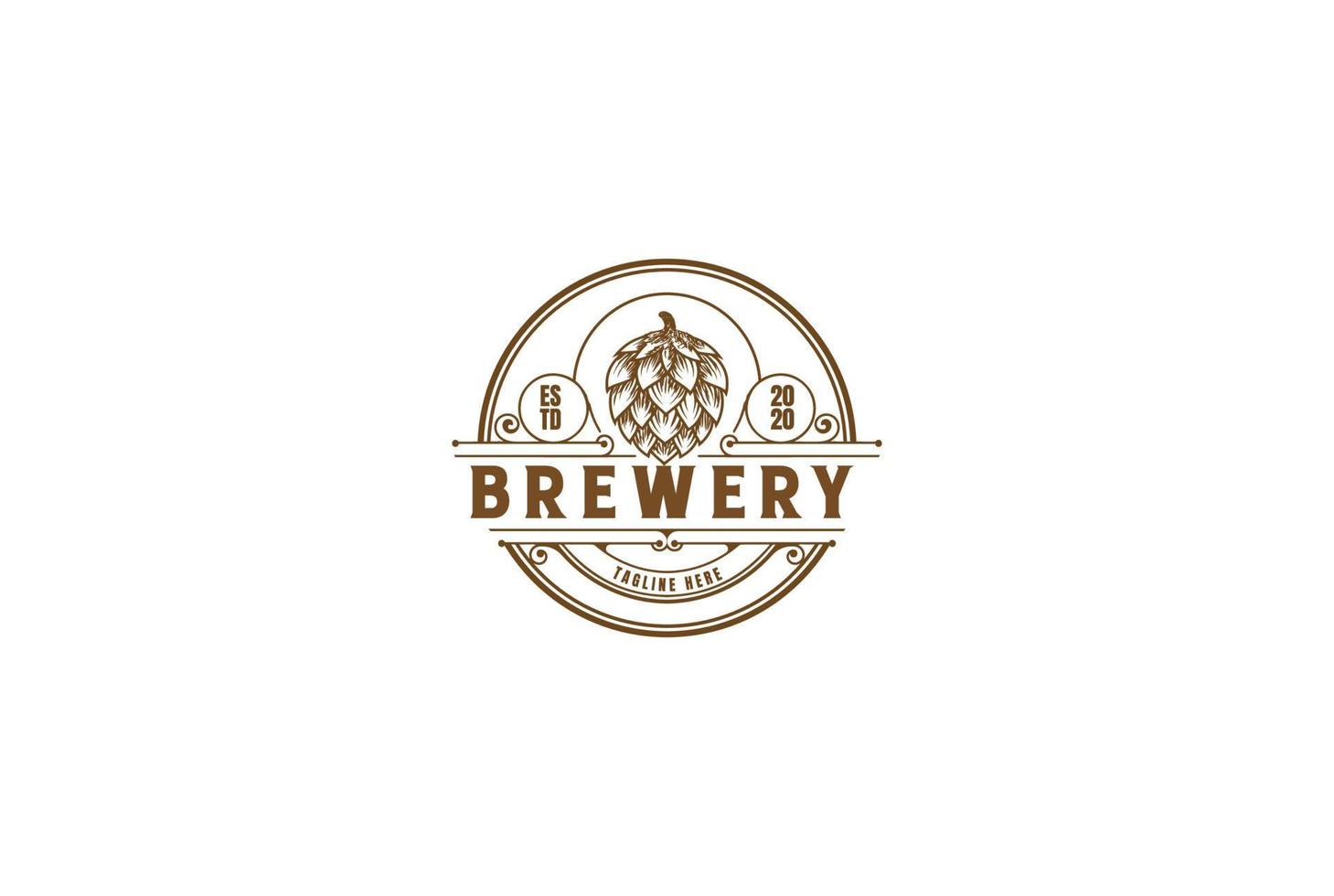This illustration features a detailed, circular logo designed for a brewery. The logo is predominantly brown against a white background. Central to the logo is an inverted plant resembling a hop, with its topmost stem pointing downward. Encircling the hop are two concentric semicircles. To the left of the hop, within the outer circle, is a smaller circle containing the letters "ESTD", and to the right is a similar circle inscribed with "2020". Below the hop, two straight lines frame the word "BREWERY" in bold, blocky print. Beneath this, another semicircle contains the placeholder text "Tagline Here," suggesting customization possibilities for businesses. This minimalist, versatile design does not include any contact details or additional information, emphasizing the logo's primary branding elements.